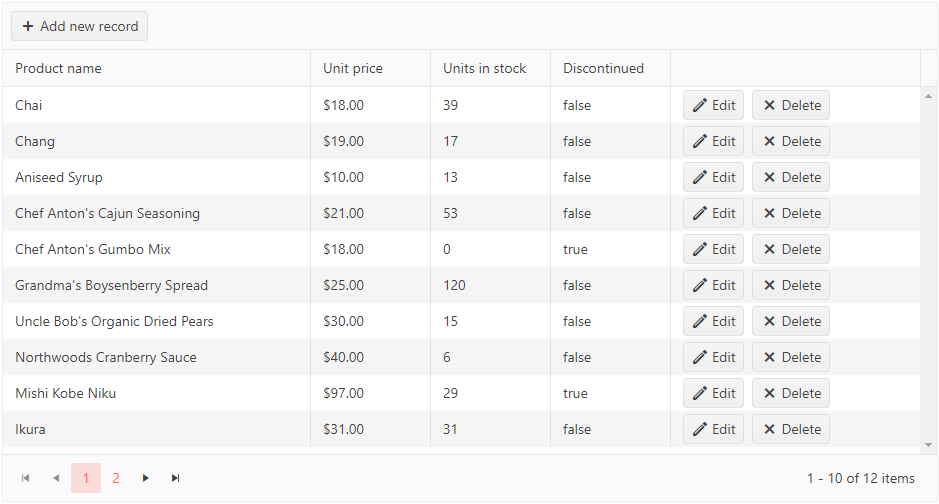The image features a user interface with a grey button located at the top left corner labeled "Add New Record." The text throughout the image is in black. Below the button is a table with five columns titled: "Product Name," "Unit Price," "Unit Stock," "Discontinued," and an action column with "Edit" and "Delete" buttons for each row. The action buttons are also grey.

The table lists the following products and details:
1. **Chai** - Unit Price: $18, Stock: 39, Discontinued: False
2. **Chang** - Unit Price: $19, Stock: 17, Discontinued: False
3. **Aniseed Syrup** - Unit Price: $10, Stock: 13, Discontinued: False
4. **Chef Anton's Cajun Seasoning** - Unit Price: $21, Stock: 53, Discontinued: False
5. **Chef Anton's Gumbo Mix** - Unit Price: $18, Stock: 0, Discontinued: True
6. **Grandma's Boysenberry Spread** - Unit Price: $25, Stock: 120, Discontinued: False
7. **Uncle Bob's Organic Dried Pears** - Unit Price: $30, Stock: 15, Discontinued: False
8. **Northwoods Cranberry Sauce** - Unit Price: $40, Stock: 66, Discontinued: False
9. **Mishi Kobe Niku** - Unit Price: $97, Stock: 29, Discontinued: True
10. **Ikura** - Unit Price: $31, Stock: 31, Discontinued: False

Each product entry has corresponding "Edit" and "Delete" buttons. At the bottom right of the table, there is a note indicating "1 to 10 of 12 items."